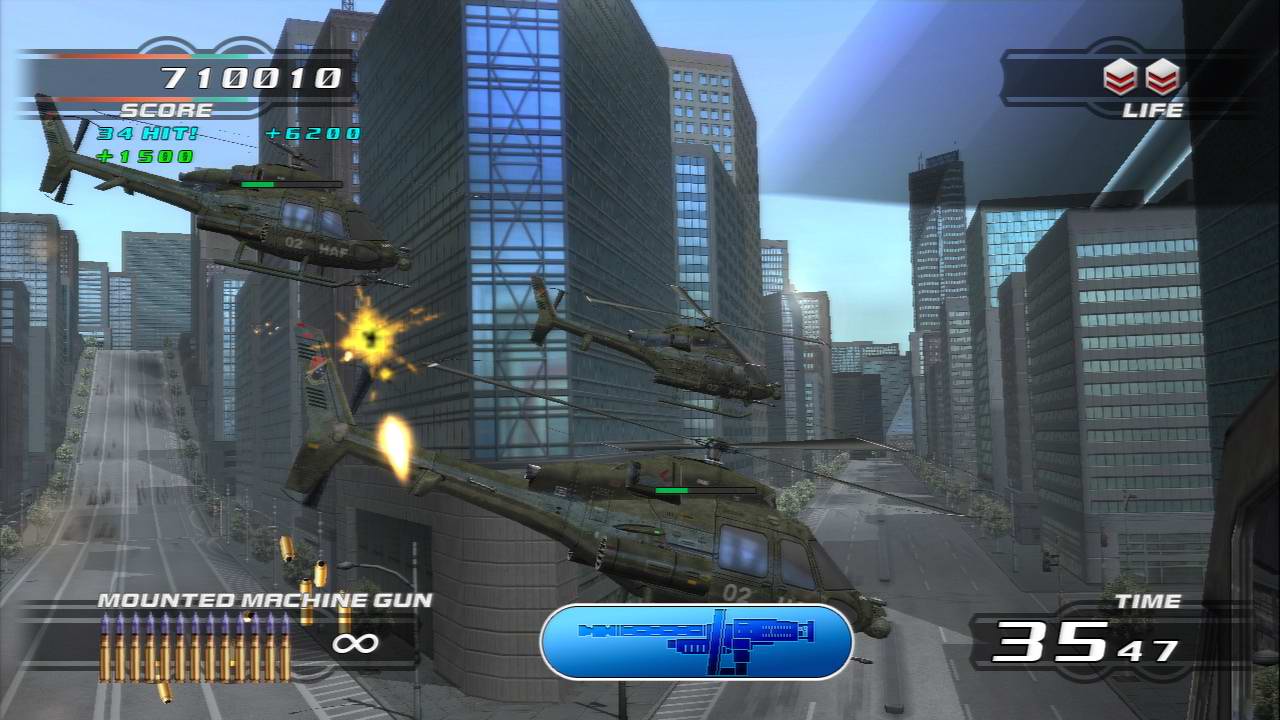This screen capture from an action-adventure game showcases an intense urban battle scene. The time stamp on the lower right corner indicates that 35 minutes and 47 seconds either remain or have elapsed in the game. Dominating the center bottom of the image is a prominent blue pill-shaped object with a darker blue gun icon facing left, possibly indicating the current weapon status.

Three attack helicopters can be seen flying amidst a cityscape filled with towering skyscrapers and reflective glass windows. The helicopters, which are approaching from the left side, add to the airborne chaos. Between the two nearest helicopters, a massive explosion lights up the sky, highlighting the high-stakes action unfolding.

Converging towards the lower center of the screen are two streets—a three-lane and a two-lane road—meeting at an angle, adding depth to the urban environment. The upper left corner displays an impressive score of 710,010 points. In the upper right, a life indicator bar shows that the player has two lives remaining, denoting the urgency of conserving health. 

In the lower left corner, the weapon status reveals a mounted machine gun in use along with the remaining ammunition count, reinforcing the tactical elements of the gameplay. This detailed scene captures a pivotal moment in the game, rich with action and strategic challenges.